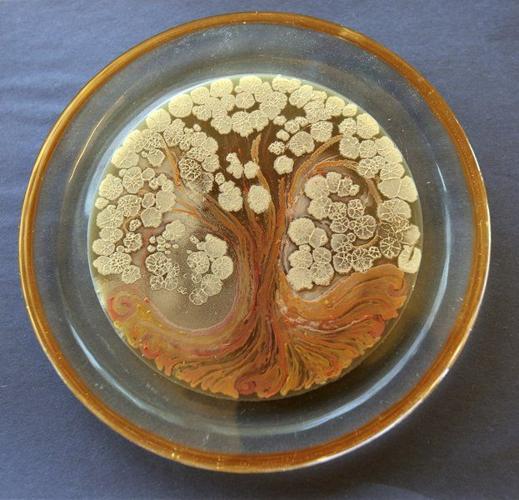The detailed description of the image reveals a unique art project, resembling an older, circular object that hints at being a coaster, carefully placed on a striking dark blue surface, possibly a tablecloth or sheet of paper. This piece, with an outer rim of golden brown and an inner section of clear plastic or glass, showcases an intricate design at its core. The design features a brown tree, complete with roots, a trunk, and branches that extend outward. Distinctive white flowers adorn the tree's branches, predominantly at the top, left, and right sides, contributing a contrast to the absence of green foliage. The overall craftsmanship suggests multiple artistic elements, with the transparent segment within the circular boundary emphasizing the tree motif. The ambient setting, enhanced by natural lighting, underscores the clarity and brightness of the image, making each component of the artwork vivid and detailed.